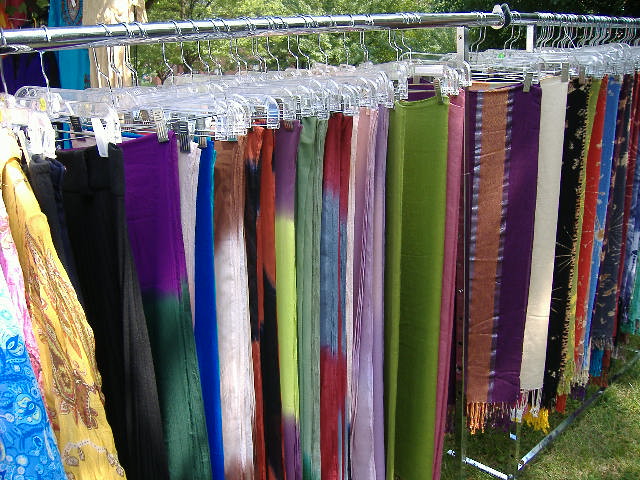This outdoor photograph captures two tall, narrow garment racks positioned side by side, each filled with an array of colorful fabrics and garments hanging neatly from clear plastic clip hangers. The scene is set on a grassy lawn, illuminated by sunlight, giving a clear indication that this image was taken outdoors. Behind the racks, we can discern some trees, bushes, and a hint of what may be a doorway under a blue sky, reinforcing the outdoor setting. The garments displayed are vibrant and varied, including solid-colored and patterned items in shades of blue, yellow, green, purple, black, white, and brown. Some fabrics showcase tie-dye designs, stripes, and symbols, with a few adorned with fringes and tassels, adding to the eclectic mix. The presence of additional shirts and garments in the background, possibly inside a tent or booth, suggests that this photograph was taken at an outdoor market.